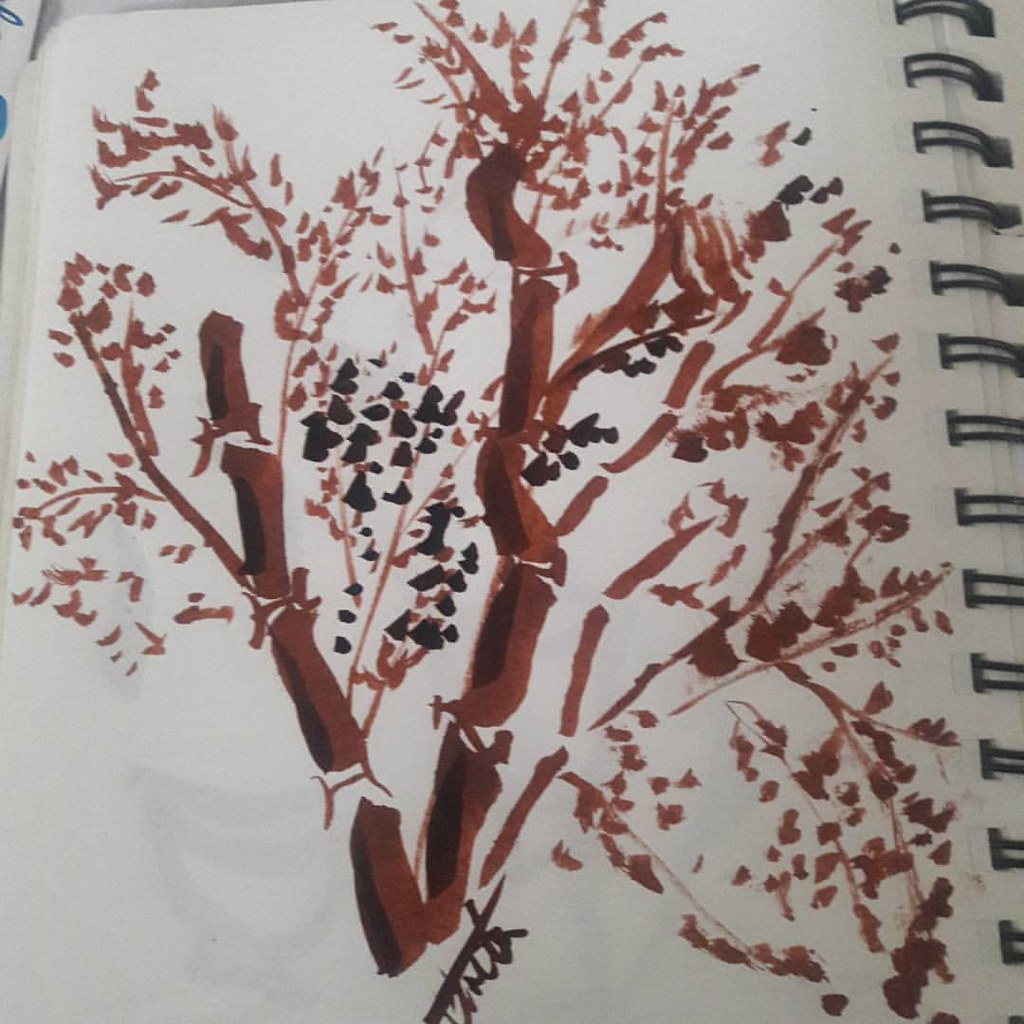This image captures a detailed view of an artwork situated within a spiral-bound notebook. The black metal spirals of the notebook are prominently visible, with a substantial number of pages turned over in the upper left corner, indicating the involvement of previous works. The artwork itself is a thoughtful painting executed using a restricted palette of dark brown, light brown, and black.

Central to the composition are the tree branches, primarily painted in light brown, featuring delicate shades of dark brown as highlights to enhance their dimensionality. The leaves adorning these branches are depicted in a sporadic pattern; primarily in light brown, they appear as though the artist lightly tapped their tool of choice—possibly a marker—creating a textured, natural effect. Among these lighter leaves, darker splotches intermingle, adding depth. These dark elements, which could be interpreted as leaves or perhaps even birds, enhance the visual intrigue and complexity of the scene.

On closer inspection, the bottom portion of the drawing reveals what appears to be the remnants of a signature, marked by scribbled lines and distinguishable characters resembling an "M" and a "Q." This hint of an artist's mark subtly underscores the authenticity and personal touch inherent in the artwork.